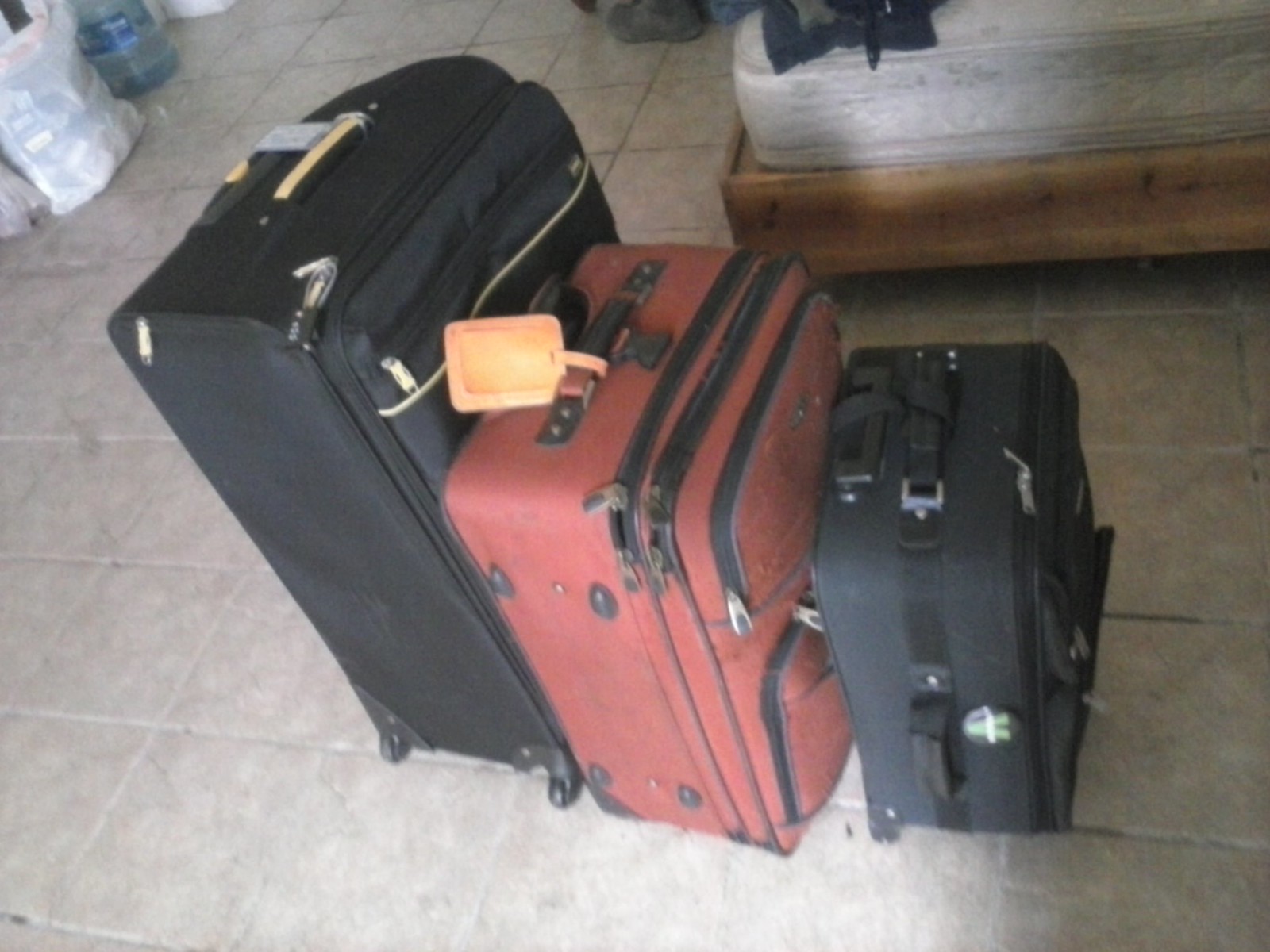In the image, three wheeled suitcases are lined up vertically on a stone-tiled floor near a bed with a wooden frame and a bare white mattress. The suitcases vary in size: the largest is black, positioned furthest back; the medium one is red, situated in the middle; and the smallest, at the front, is also black. Each suitcase features travel tags for identification, and they all appear zipped up and packed. There is also some additional clutter in the scene, including a white trash bag filled with items and a five-gallon blue water bottle. Based on this setup, it seems this family is ready to move or depart soon. No people are present in the frame.